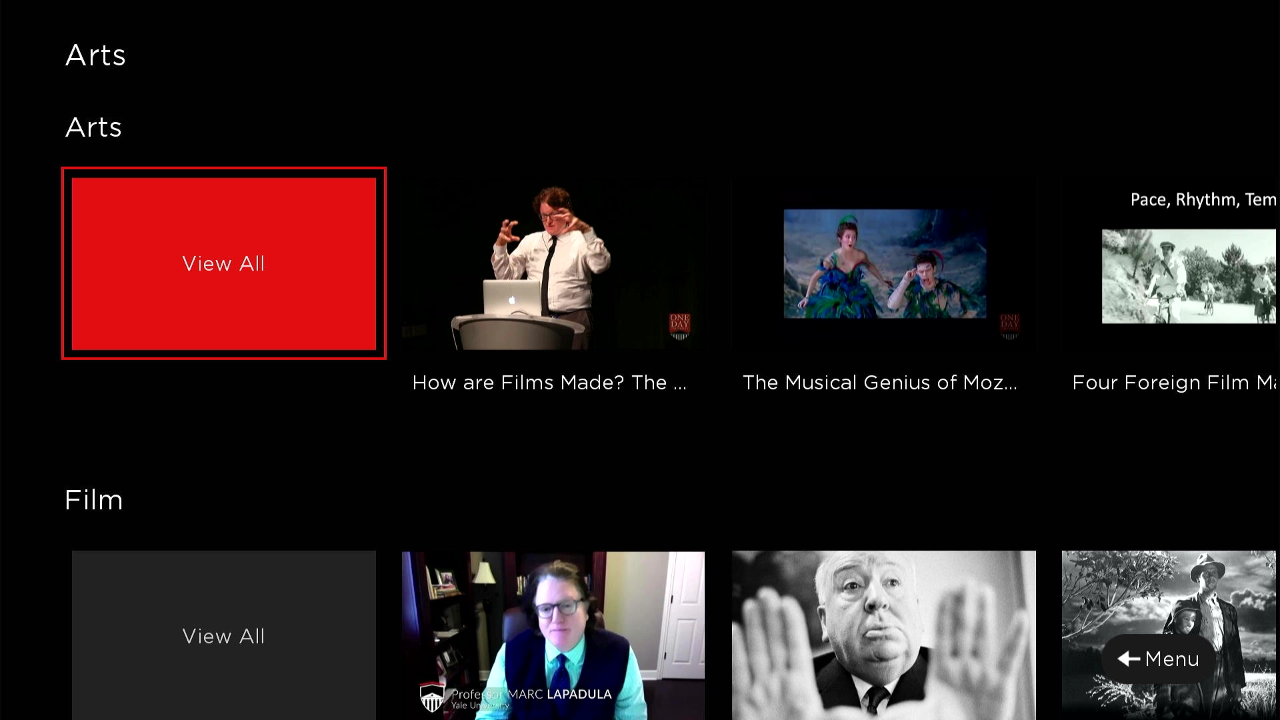The image features a stark black background with prominent text elements in contrasting colors. At the top, in refined white text, the word "Arts" appears with a capital A, and directly below it, the word "Arts" is repeated in a smaller font size.

Dominating the center is a solid red square with a red border, contrasting against the black interior. Inside this square, the phrase "View All" is inscribed in white, utilizing capital letters for "V" and "A."

The image also showcases several text snippets associated with various themes:

- "How are films made?" is one line, accompanied by an incomplete phrase starting with "the..."
- Another snippet reads, "The musical genius of M-O-Z..." indicating a mention of Mozart.
- There is an incomplete title starting with "pace, rhythm..." followed by a truncated "T-E-M," and beneath it, the partial phrase "For a Foreign Film," with a cut-off capital M.

At the bottom, the word "Film" is displayed in white text with a capital "F," encased within a lighter black box. This box also features the "View All" prompt, again in white with capital letters for "V" and "A."

There are two prominent images:
1. A person inside a room, identified as Professor Mark Lapadula (spelled out as L-A-P-A-D-U-L-A). This individual bears a resemblance to Alfred Hitchcock.
2. A black-and-white image of a person with trees in the background. This image includes a banner featuring a left arrow key and the word "Menu."

Overall, the combination of text and images creates a rich, multi-layered visual narrative focused on various aspects of film and the arts.